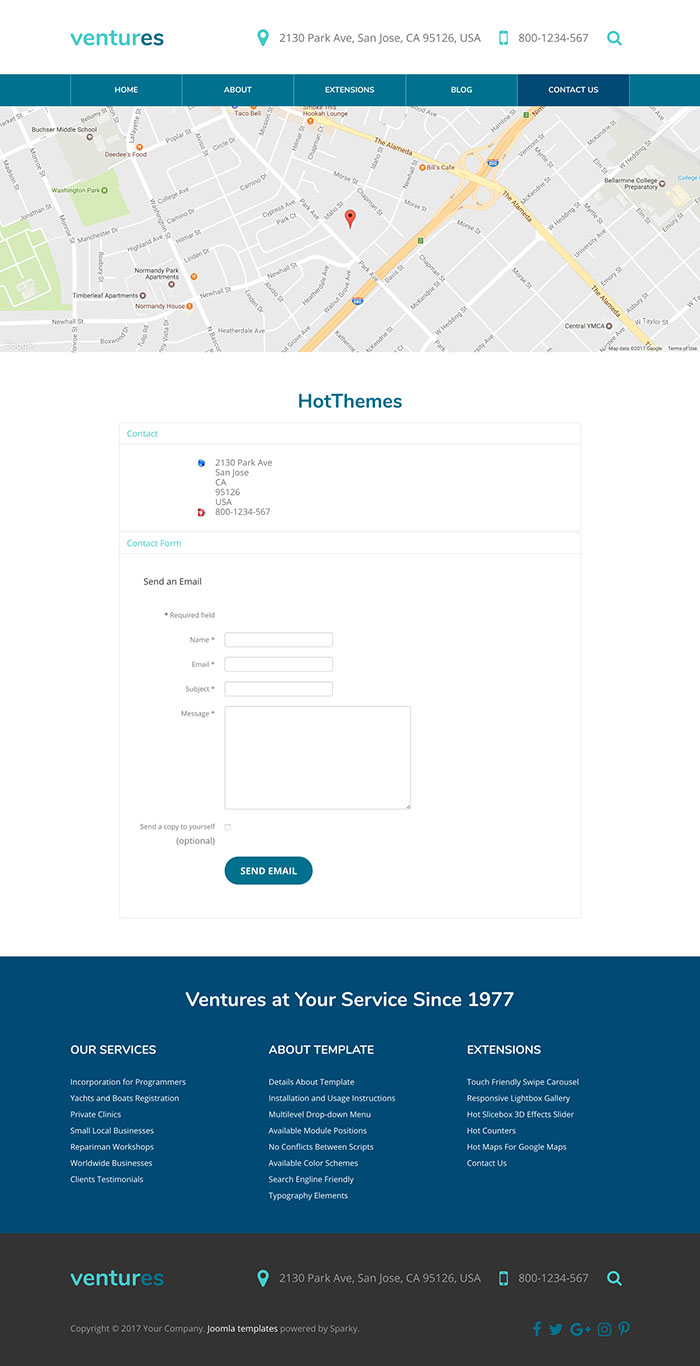**Company Webpage Screenshot Description**

The image depicts a company webpage for "Ventures." At the top of the page, the company name "Ventures" is rendered with the letters "V-E-N-T-U-R" in cyan blue and the letters "E" and "S" in dark blue. Below the company name, there's an icon of a cyan blue pin followed by the address "2130 Park Avenue, San Jose, California, 95126, USA," written in black with "Avenue" abbreviated as "AVE." Adjacent to this, a cyan blue phone icon is visible with the phone number "800-1234-567" in black, and a cyan blue magnifying glass icon is positioned nearby.

Embedded in the design is a gray map with green, orange, and yellow areas, surrounded by a dark blue bezel containing clickable buttons separated by white borders. These buttons include, from left to right, "Home," "About," "Extensions," "Blog," and "Contact Us," with the latter appearing in a very dark blue hue. At the bottom of the map, the text "Hot Themes" appears in dark blue.

Below, there's a rectangular section divided into several parts. On the left, in cyan blue, the word "Contact" appears, leading to a mostly white empty section on the right. There's also a blue box with some cyan elements listing "2130 Park Avenue, San Jose, California, 95126 USA," and a red image against a white background displaying the phone number "800-1234-567." Below it is "Contact Form" in cyan blue. The form features fields for "Send an Email" in black, with notes indicating required fields marked by an asterisk. Fields include "Name," "Email," "Subject," and "Message," each with corresponding input boxes. Additionally, there's an optional checkbox labeled "Send a Copy to Yourself." A dark blue oval button with bold white text labeled "Send Email" is positioned at the bottom of the form.

Beneath, in dark blue and bold white text, the phrase "Ventures at Your Service Since 1977" is displayed. Alongside, the headings "Our Services," "About Template," and "Extensions" are outlined, offering details on various services and template features.

At the bottom left of the webpage, within a dark black bezel, the company name "Ventures" is repeated, with the letters "E" and "S" in dark blue. Following the company name is a cyan blue pin icon and the address "2130 Park Avenue, San Jose, California, 95126, USA" in gray. Another cyan blue phone icon is shown with the number "800-1234-567" listed in proximity. Below this is a cyan blue magnifying glass icon.

On the left, the footer text includes "Copyright @ 2017 Your Company," "JOOMIA Templates" in white, and "Powered by Sparky" in dark gray. Adjacent to this are dark blue clickable buttons featuring logos for Facebook (an F), Twitter (a tweeting bird), Google Plus (a G with a plus), Instagram (a rounded square with a circle), and Pinterest (a curly P).